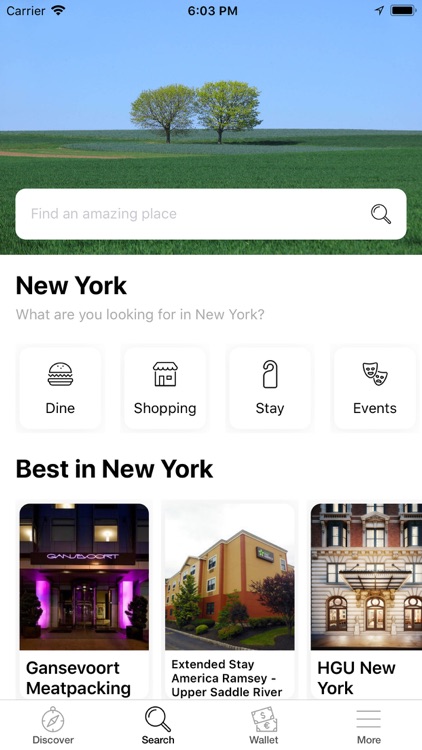This is an app screenshot featuring a travel-related interface. At the top, there is an image of a verdant field dotted with two prominent trees. Directly beneath the image, a search bar is prominently displayed with the placeholder text "Find an amazing place" alongside a magnifying glass icon for searching. The main heading "New York" is presented in bold, black text. Below it, a prompt reads "What are you looking for in New York?" accompanied by four white square buttons, each adorned with representative icons: a cheeseburger for dining, a shopping bag for retail, a door hanger for accommodations, and theater masks for events.

The lower section titled "Best in New York" showcases three images, presumably of notable buildings or hotels. The first image depicts "Gansevoort Meatpacking," the second highlights "Extended Stay America, Ramsey, Upper Saddle River," and the third features "HGU New York."